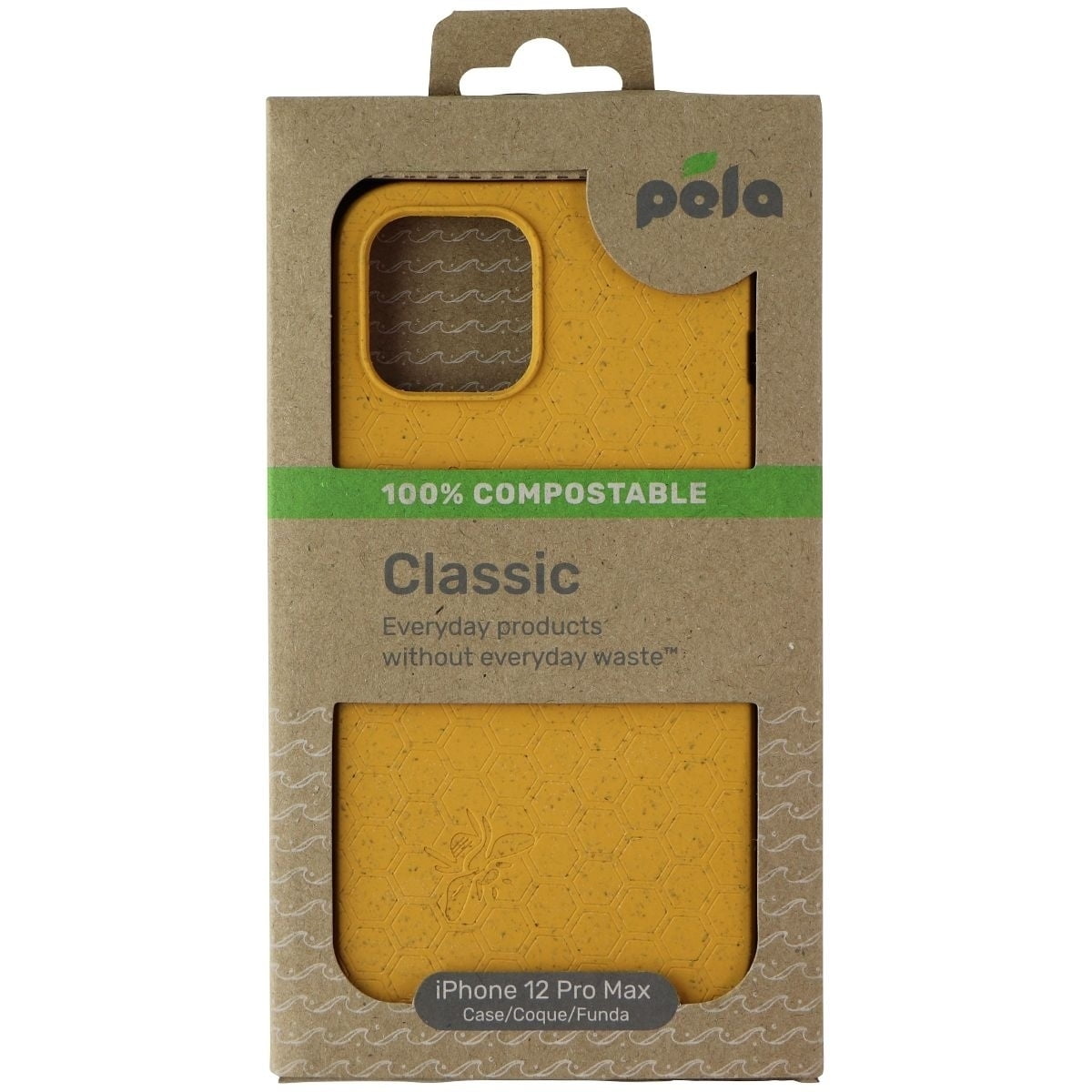The image depicts sustainable packaging for an iPhone 12 Pro Max case by Kella. The phone case, enclosed in brown cardboard with a small hook for hanging, is clearly visible through the packaging. The cardboard container features a notable bright green stripe with white text stating "100% compostable" and gray letters underneath that say "classic, everyday products without everyday waste." The brand name "Kella" appears in the upper right corner, marked by a green leaf over the letter 'E'. The mustard yellow phone case inside has a distinct honeycomb or hexagonal pattern, along with an embossed illustration of a bee, reinforcing its eco-friendly theme. Translations for "case" in other languages (such as "caulk" and "funda") are also present on the packaging, further adding to its detailed design.